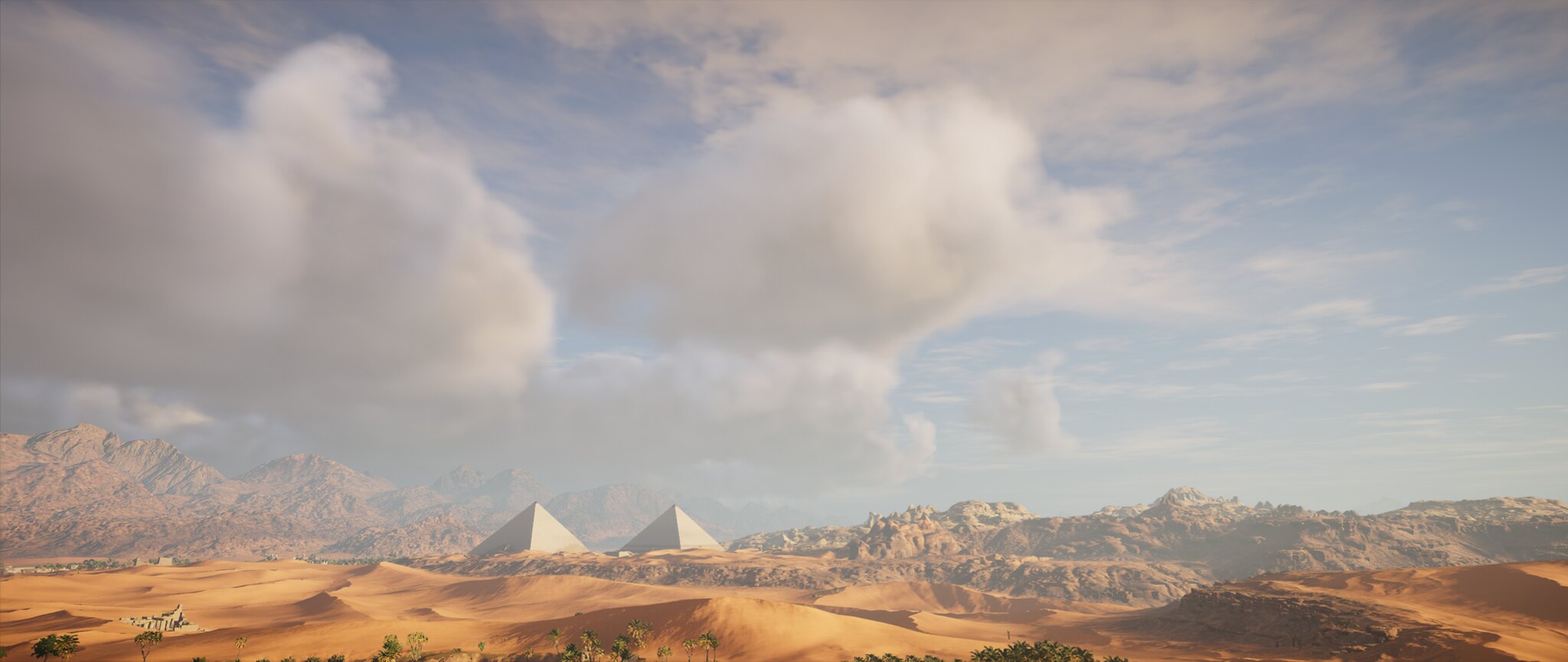In this captivating outdoor image, possibly a photograph or painting, we are presented with a desolate, desert-like landscape set in a long rectangular frame. The sandy foreground is composed of undulating hills and sand dunes, showing shadows and adorned with golden dried grass. To the right, the colors shift to the reds and blues reminiscent of the Badlands of South Dakota.

Prominently situated just left of center are two small, white pyramids that appear starkly out of place amid the rugged terrain. These pyramids stand closely together against a backdrop of darker brown hills, with rough, rocky mountains extending to the left. On the right, shorter, rocky areas contribute to the overall ruggedness of the scene.

Above, the sky takes up approximately two-thirds to three-quarters of the image, featuring a beautiful gradient of blue with puffy white and grey clouds scattered more densely to the left. The serene, expansive sky contrasts strikingly with the harshness of the wasteland below, accentuating the surreal and otherworldly feeling of the landscape.